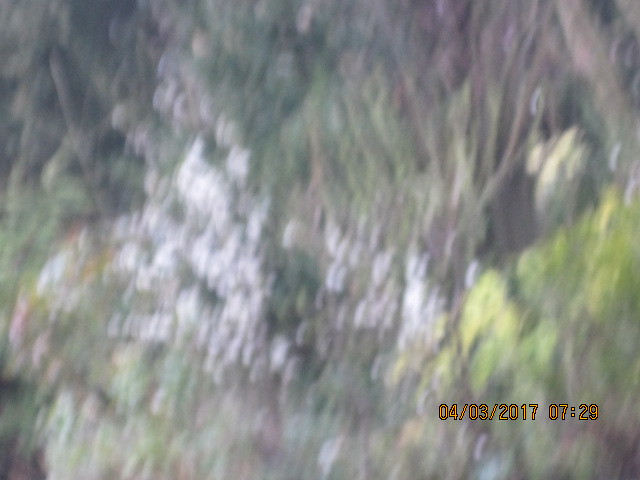This is a super blurry aerial photograph, seemingly taken from a drone, capturing an overhead view of a wooded area. The center and slightly to the left showcase clusters of white patches that resemble flowers of a plant, despite the blurry quality. On the right side, there are noticeably brighter green trees, contrasting with the rest of the foliage. In the upper left corner, the image appears to depict a collection of sticks and twigs. The photograph is timestamped with the date 04-03-2017 at 07:29.